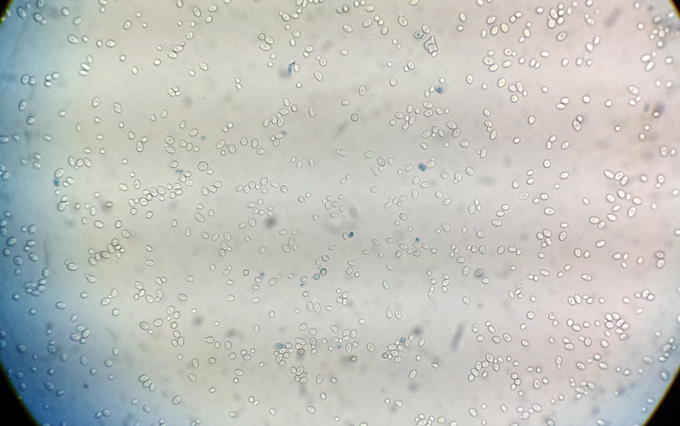This image, likely taken through a microscope, displays a detailed view of a scientific specimen. Dominating the center is a large, nearly perfectly round white sphere, which stretches beyond the edges of the rectangular frame, causing the sides of the image to blend into the black corners. Within this central sphere, hundreds of tiny white dots are dispersed without any specific pattern, reminiscent of bacteria or cells magnified under laboratory conditions. Interspersed among these white dots are darker spots, some nearing black, creating contrast. On the left side of the image, there is a subtle blue hue, perhaps a reflection or shadow cast by the microscope’s light. The overall color palette is muted, featuring off-white, gray, and dark-gray tones. This intricate setup suggests a meticulously colored scientific sample aimed to highlight minute details for clearer observation.